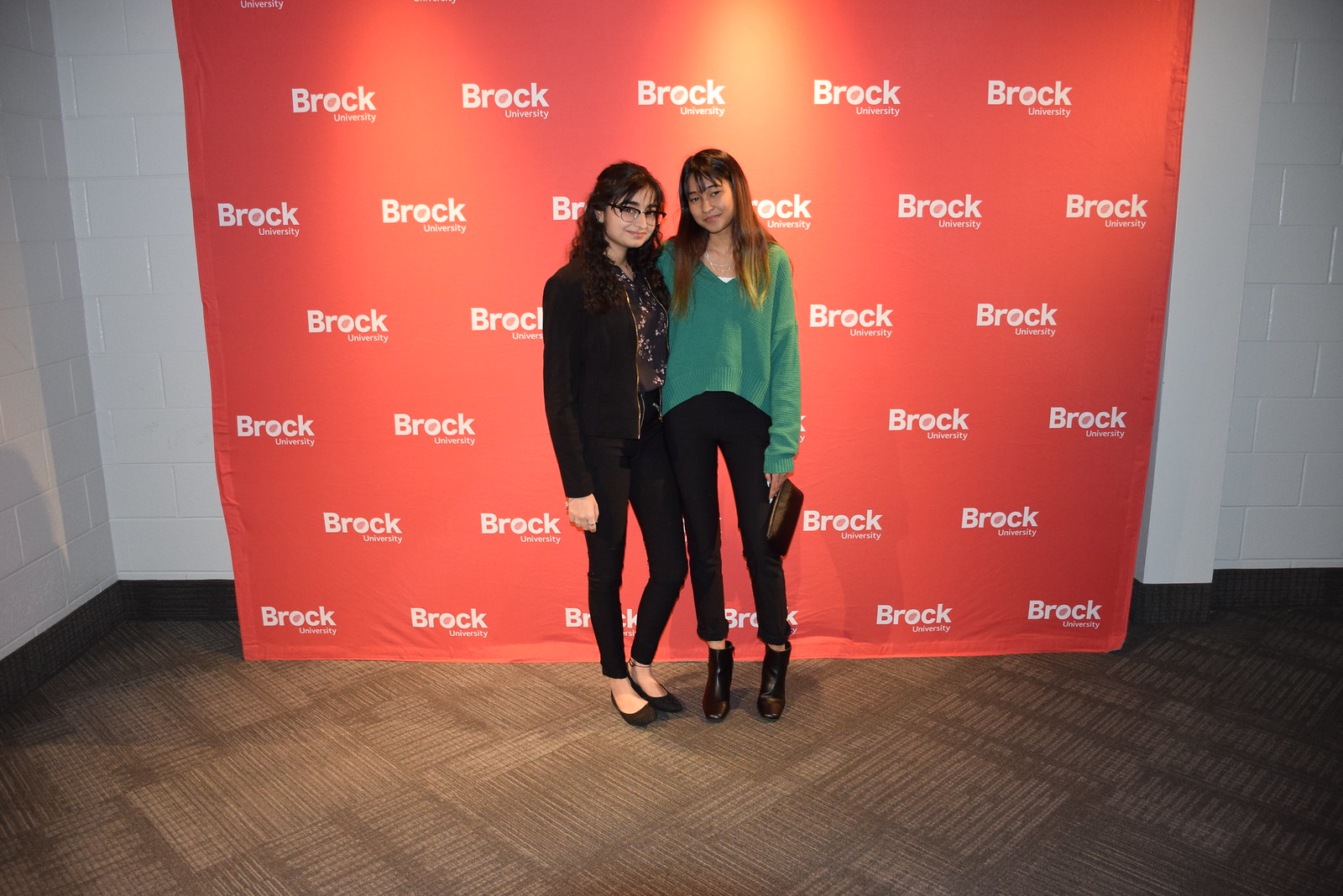This is a photo of two young women standing in front of a large red banner that repeatedly reads "Brock University" in white. The banner is set against a white stone or concrete wall, typical of a school or university setting, and the floor seems to be either brown tile or a carpet mimicking a tiled design. Both women are posing for the camera, smiling and standing close together.

The woman on the right, who appears to be of Asian descent, has long, light brown hair flowing over her shoulders. She is wearing an oversized green sweater layered over a white top, paired with black pants and brown high-heeled boots. She's holding a small clutch in her left hand.

The woman on the left, who has dark, curly hair and is of possible South Asian descent, is wearing glasses and is dressed entirely in black. Her attire includes a well-designed black shirt, a black jacket, black trousers, and black heeled shoes. She has some rings on her fingers and a black thread on her left ankle. The two women have their arms around each other's backs, indicating a close and friendly relationship.